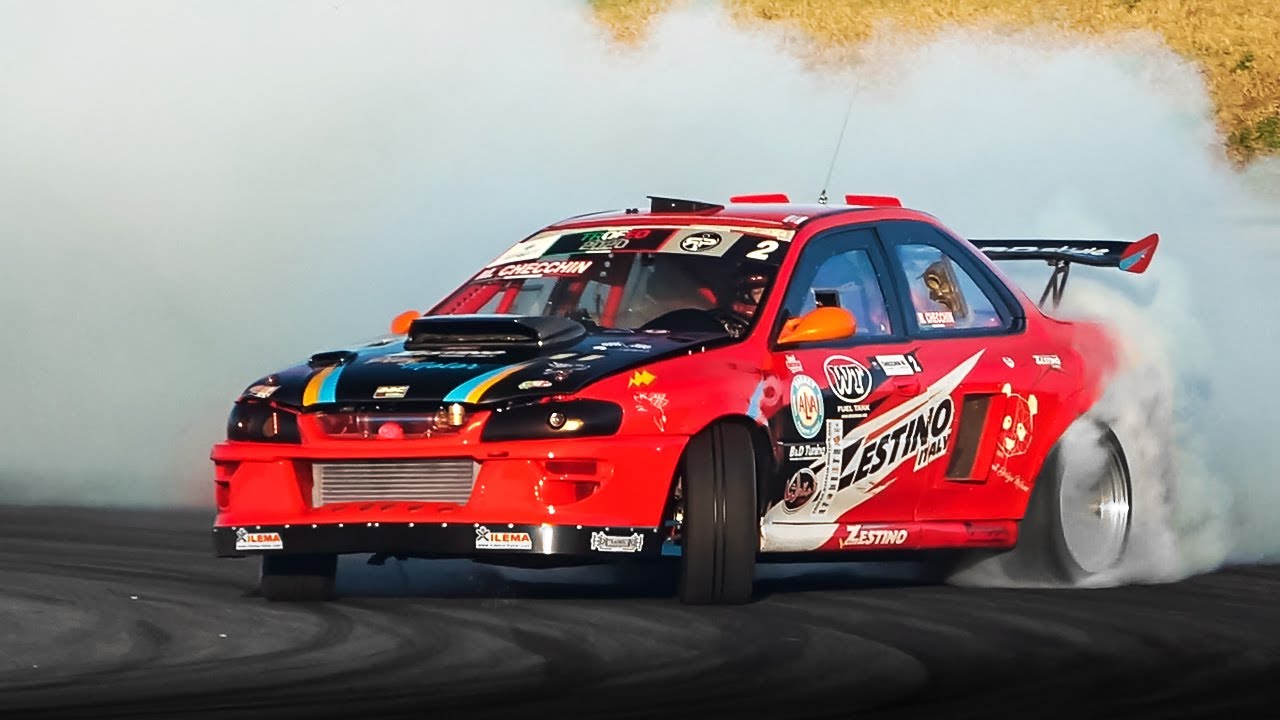The photograph captures an exciting action shot of a professional red and black race car, likely engaged in drifting or performing a burnout on a dark asphalt racetrack. The car, which features a bold "Zestino" logo in black and white lettering along its sides, is slightly sideways with its front wheels turned, and thick white smoke billowing from its spinning back tires. This custom-built race car, which may resemble a Subaru sedan, boasts a black hood with blue and yellow stripes, slightly tinted windows, and numerous advertisement stickers, including AAA, WT, Xilema, and Chechen. The passenger-side door exhibits white splotches. The car features a rear spoiler, orange side mirrors, and a visible driver through the windshield. The background is filled with smoke, but patches of a yellowing grassy area can be seen. Tire marks curve around the black tarmac, indicating the car's path, and enhancing the dynamic nature of this thrilling moment.